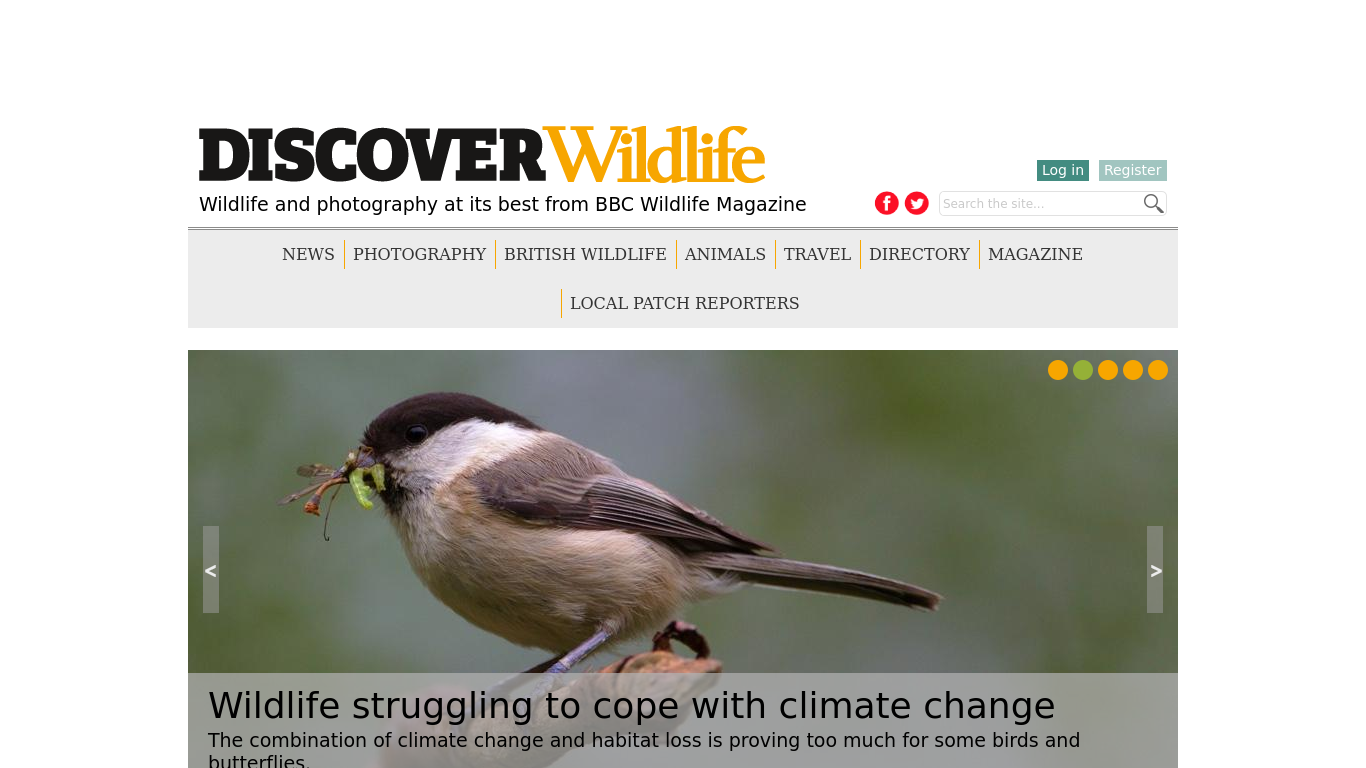Title: "Bird with Grasshopper Highlights Climate Change Challenges in BBC Wildlife Magazine"

Caption: The vibrant cover of an online edition of BBC Wildlife Magazine showcases the stunning beauty and complexity of wildlife photography. Central to the image is a small brown bird, perched delicately on a slender branch. This avian subject, characterized by its short wings, rounded belly, and distinctive black crown with contrasting white crest, gazes intently. In its beak, the bird clutches a grasshopper, emphasizing the daily survival challenges wildlife faces. The magazine’s header, "Wildlife Struggling to Cope with Climate Change," underscores the urgent narrative.

The interface of the digital magazine, likely viewed on a tablet, displays an array of clickable sections such as News, Photography, British Wildlife, Animals, Travel Directory, and Magazine Local Patch Reporters. Navigation arrows on either side of the image allow readers to seamlessly explore accompanying stories and photographs, enhancing the immersive experience. This particular image is positioned as the second feature in a sequence of five, inviting readers to further explore the impact of climate change on diverse species.